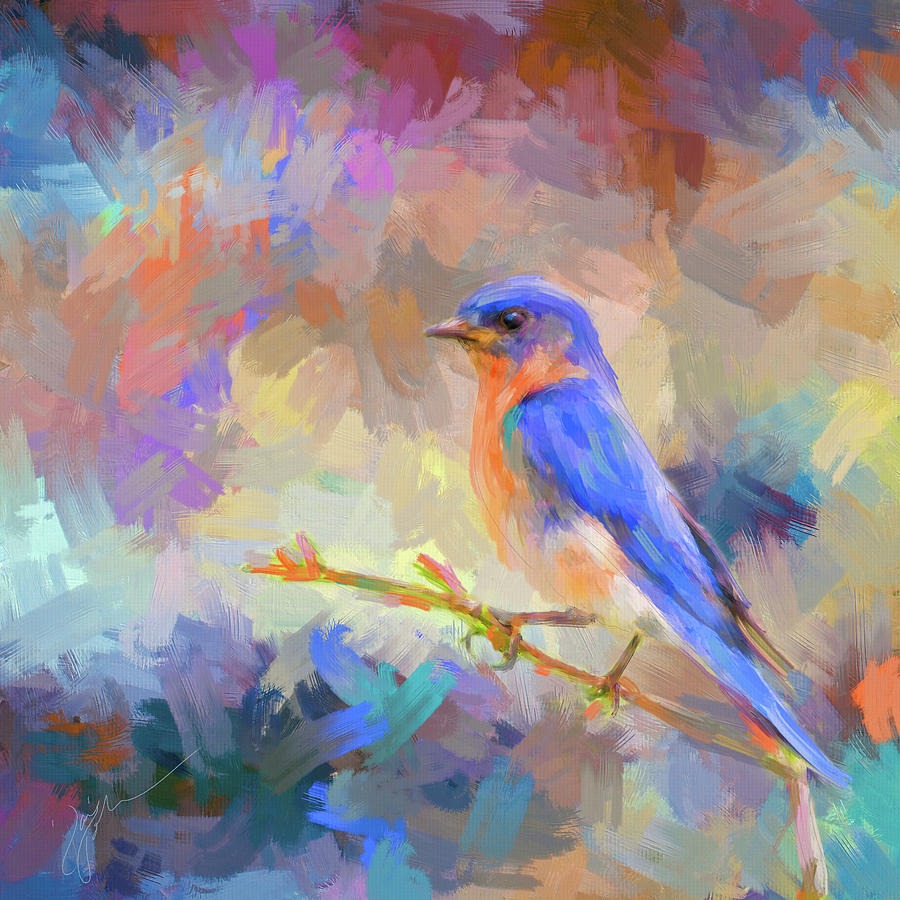This is an intricate watercolor painting featuring a vibrant bird perched on a single branch. The bird, positioned slightly to the right of the center, has a striking blend of colors: a blue back and head, transitioning into an orange breast that merges seamlessly into a cream base. The feathers are depicted with a pointed texture, and its legs and feet are painted a golden color. The bird is also marked by its black eyes and is gazing towards the left side of the painting.

The background is a mesmerizing mix of multiple colors, including blue, orange, pink, white, fuchsia, yellow, maroon, magenta, and beige, creating a fractal-like appearance. This layered, textural effect infuses the background with a sense of dynamic movement and depth. Adding a personal touch, the artist's signature, written in flourished white lettering, is located at the bottom of the artwork, though it is not easily legible.